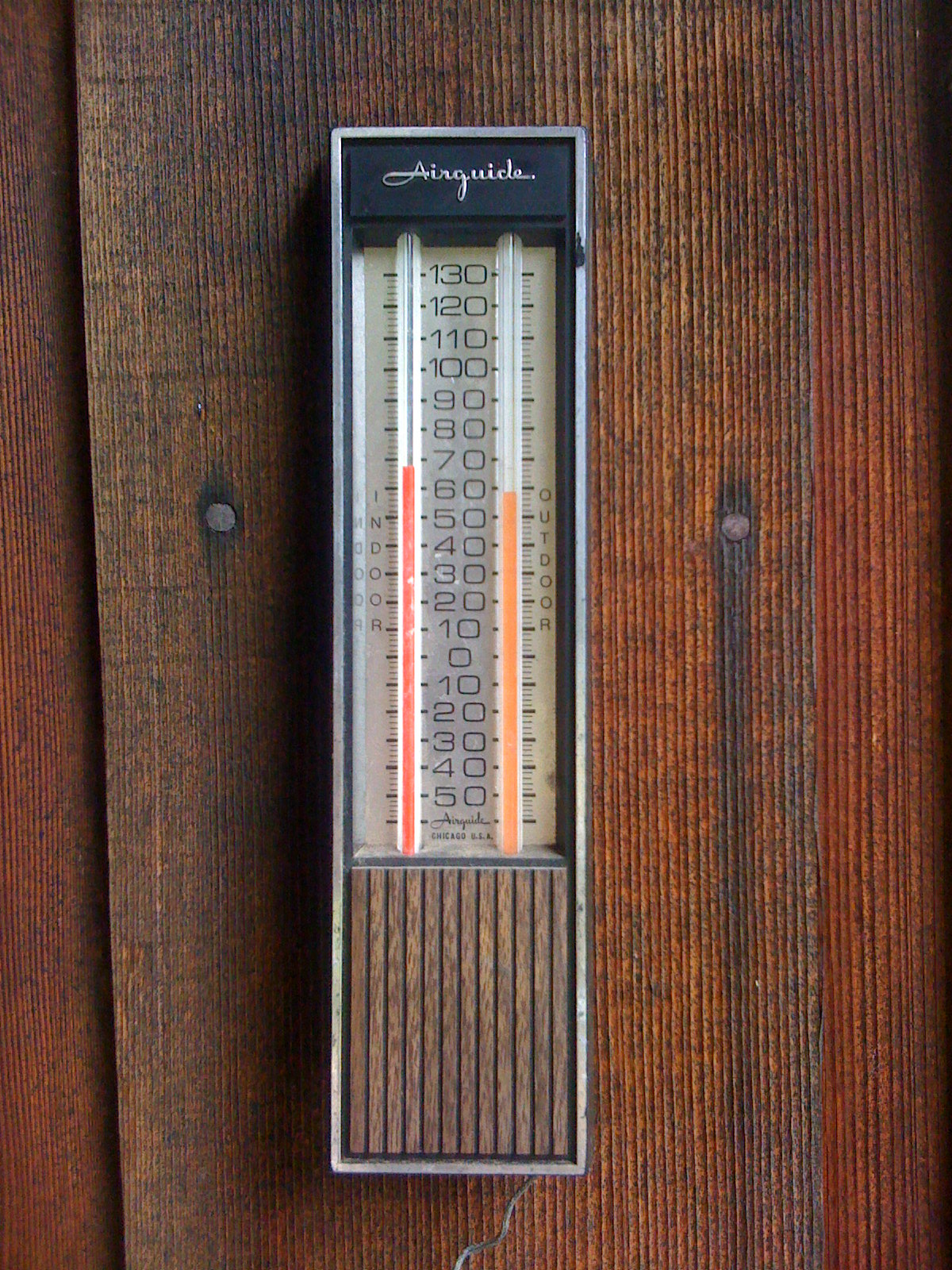This image depicts a vintage thermometer manufactured by Air Guide. The thermometer, rectangular and boxy in shape, is mounted on a wooden wall lined with thin vertical paneling. The device has protruding sides and shows signs of significant age and wear. The thermometer's base, where temperature markings are displayed, is distinctly worn out, contributing to its antique appearance. The color of the left side is a darker, reddish hue, while the right side has a lighter, more orangey shade. A noticeable yellowish tinge stains the overall structure, and faint marks can be seen on the red parts of the thermometer. In very small print on the right-hand side, the word "OUTDOOR" is visible, along with an almost illegible note possibly indicating its manufacture in the USA. A wire extends from the bottom of the thermometer, disappearing out of the frame. The entire scene is bathed in a subtle nostalgic ambiance, evoking a sense of history and bygone eras.